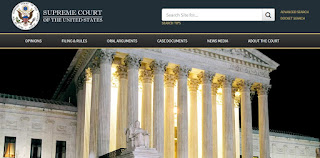A detailed image of the White House alongside the Supreme Court of the United States. The image prominently features the Supreme Court building, adorned with a badge depicting an eagle, symbolizing justice. At the top of the image is a dark blue header, below which is a search bar accompanied by a magnifying glass icon. Beneath the search bar, there is a gray rectangular section containing a list of terms in white text. Although some of the words are unclear, they appear to include categories such as "Opinions" or "Options," "Fine Arts," "Car Accidents," and possibly "New" and "About the Court." The setup suggests an official or informational context, likely pertaining to legal matters or court information.